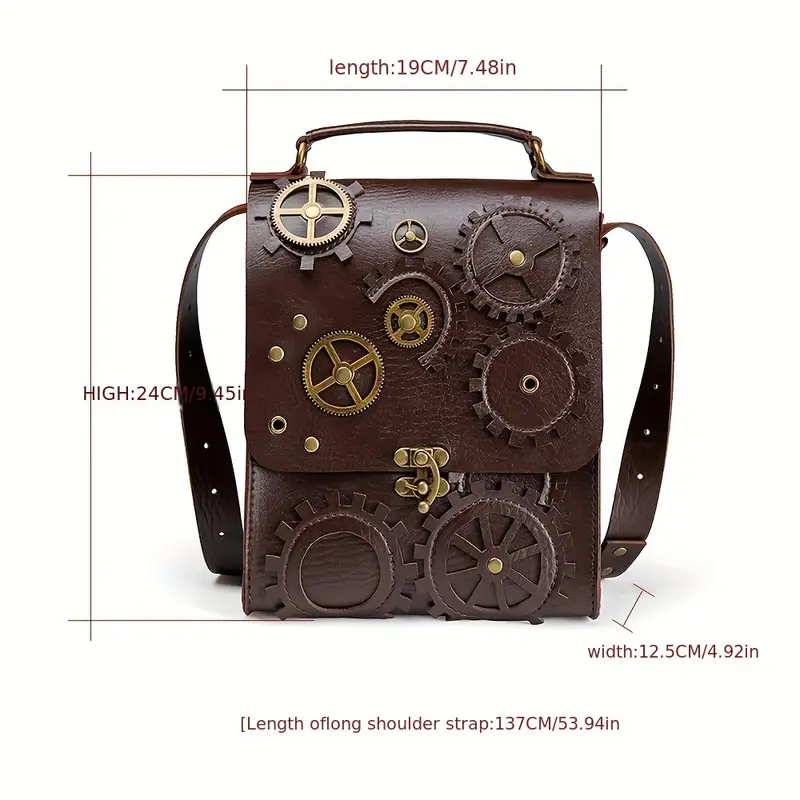The image showcases a steampunk-style leather bag positioned centrally against a white background. The bag, primarily chocolate brown in color, features a series of gold-colored cog wheels and metal gear designs, adding to its distinctively machinish aesthetic. Detailed measurements are prominently displayed: length 19 centimeters (7.48 inches), height 24 centimeters (9.45 inches), and width 12.5 centimeters (4.92 inches). The shoulder strap's length is given as 137 centimeters (53.94 inches). The bag includes gold-colored metal fastenings and a latch located in the middle of its front flap, with straps on either side and handles on top, reinforcing its steampunk motif reminiscent of vintage camera bags.